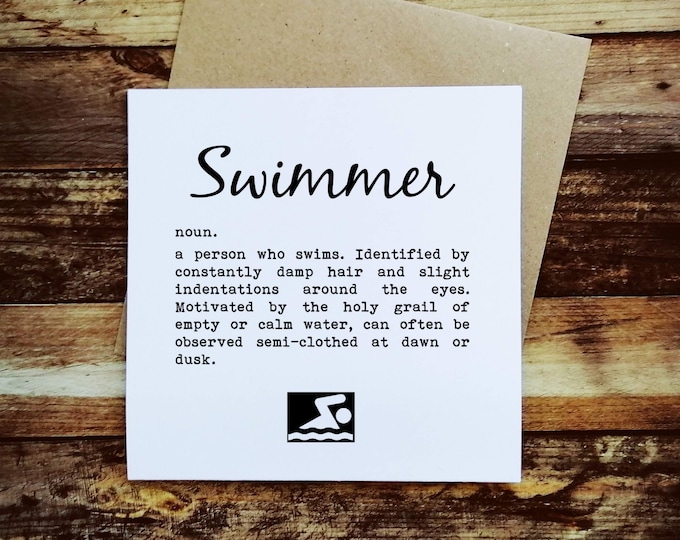The image captures a detailed photograph centered on a white card featuring black cursive text that reads "Swimmer." Below this headline, in a clear and precise font, the card defines the term as a noun, describing a "swimmer" as a person who swims, characterized by consistently damp hair and slight indentations around the eyes. Furthermore, it notes that swimmers are motivated by the quest for empty or calm water and are often observed semi-cloaked at dawn or dusk. At the bottom of the card, there's an illustration—a black square with a swimming stick figure depicted with squiggly black and white lines to represent water. This white card rests on a light brown, possibly cardboard, piece, which in turn is placed on a background made up of horizontally aligned wooden planks. These planks vary in shades from medium to dark brown, beige, and gray, suggesting a warm, rustic texture. The entire arrangement suggests a thoughtful composition with a focus on words and definition, set against the visually appealing, natural wood backdrop.